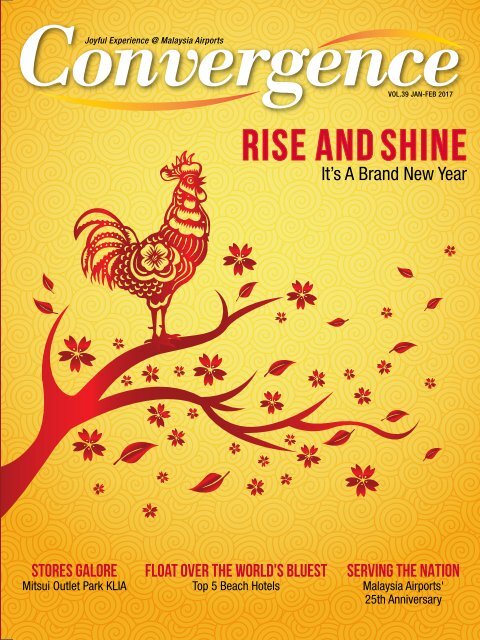This is the cover of Volume 39 of Convergence magazine, dated January to February 2017. The cover features a vibrant yellow background accented with swirling shapes. At the top, the magazine's title "Convergence" is prominently displayed in bold white lettering. Above the title, in small black print, it reads "Joyful experience at Malaysia Airport." Just below the title, in red letters, it declares "RISE AND SHINE." Beneath that, in smaller black script, it says "It's a Brand New Year."

Central to the cover is a hand-drawn rooster standing tall on a tree branch extending from the left side of the cover. The rooster and tree branch, complete with leaves and flowers, are detailed in an artistic, marker-like style, with the leaves appearing to blow off to the right.

The bottom of the cover features several article titles in red and black text. On the left, in red, "Stories Galore." Adjacent to that, in black script, "Mitsui Outlet Park KLIA." In the center, also in red, "Float Over the World's Bluest." Below that in black, "Top Five Beach Hotels." On the right, in red, "Serving the Nation." Underneath in black, it continues, "Malaysia Airports' 25th Anniversary." To the right of the title "Convergence," in small black text, it states "Volume 39 January to February 2017."